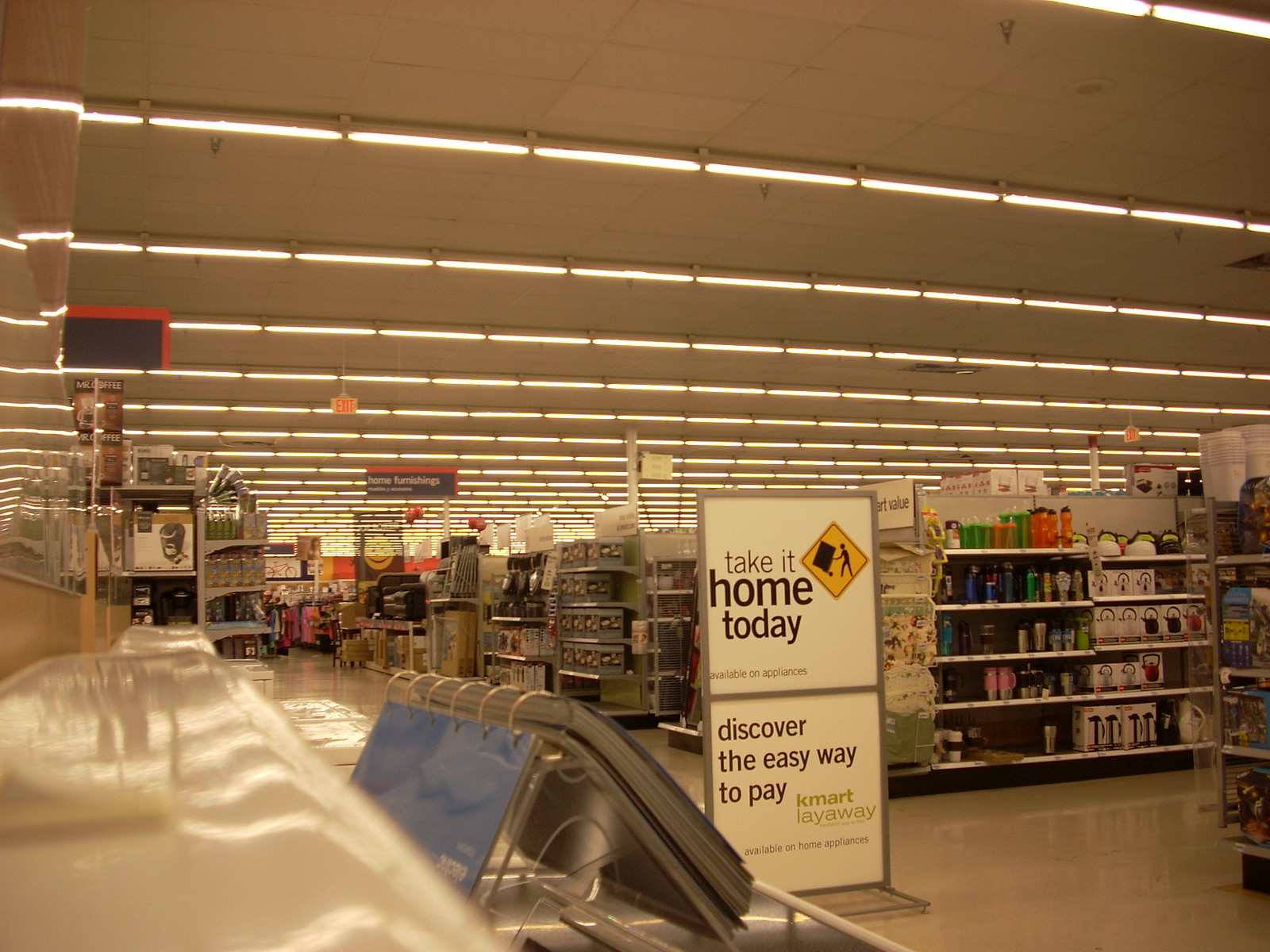This photo captures the vibrant interior of a Kmart shopping center. Overhead, gray signs outlined in orange denote the Home Furnishing section, inviting shoppers to "Take it home today" and "Discover the easy way to pay." To the right, a well-organized shelf showcases a variety of insulated travel cups and teapots, appealing to customers looking for practical kitchen and travel accessories. On the left, a calendar or spiral-bound book is prominently displayed, propped open to reveal its pages. Adding a touch of whimsy to the scene, a black flag featuring a cheerful yellow smiley face hangs from the ceiling, enhancing the store's welcoming atmosphere.